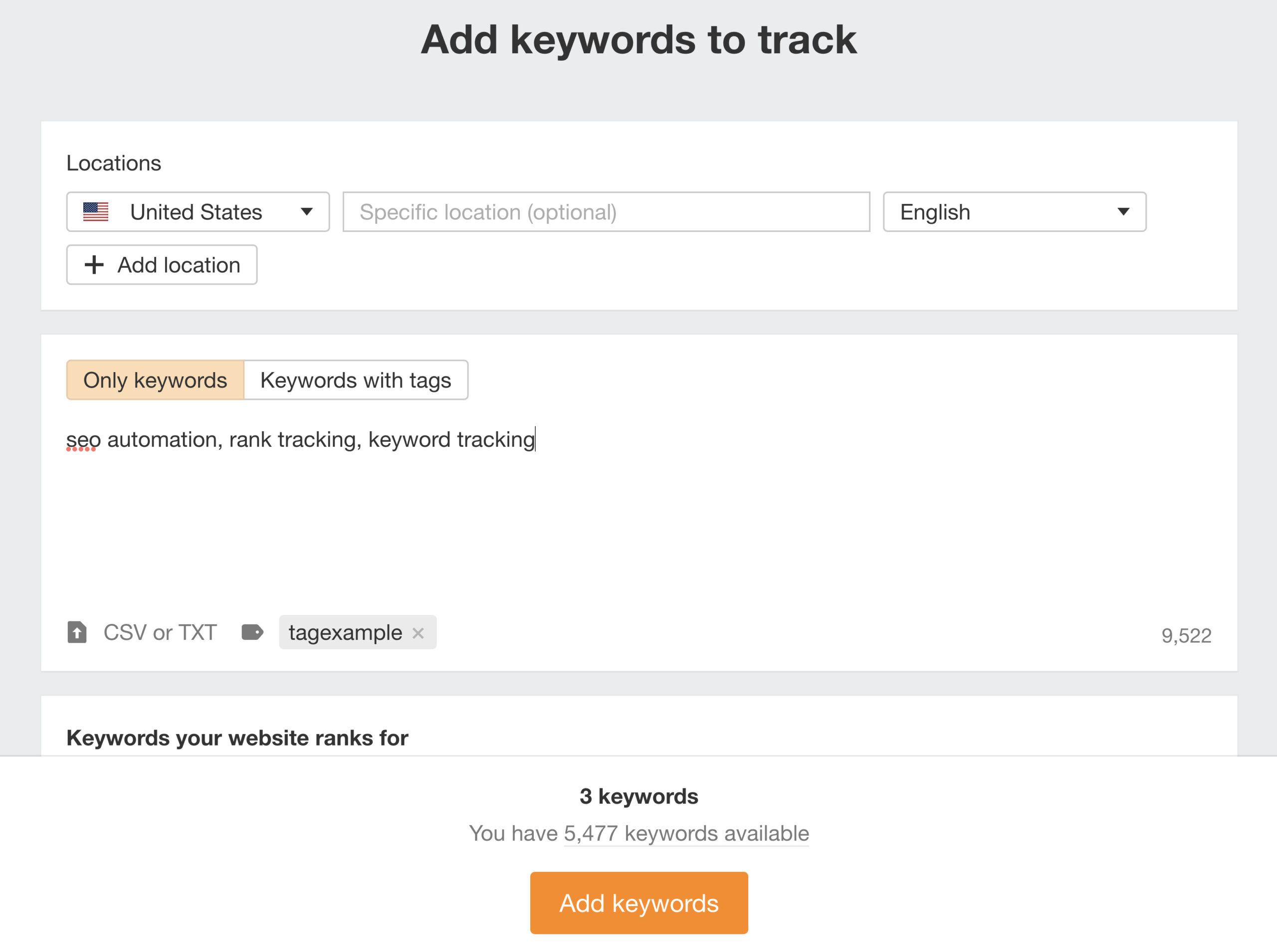In the displayed image, we see a user interface designed for adding and tracking keywords on a website. The background color of the interface is light gray, creating a subtle and clean visual appearance. 

At the top center of the interface, the title "Add Keywords to Track" is prominently displayed in black text. There are no other elements on either side of this title, keeping the focus on the main functionality.

Beneath this, there is a rectangular section labeled "Locations" at the top left. Within this section, there are three individual boxes. The first box contains the text "United States" alongside a United States flag icon to its left and a downward-pointing arrow to its right, indicating a dropdown menu. The second box is currently empty but features placeholder text in light gray, stating "Specific location" with "Optional" to its right, suggesting that location entry is not mandatory. The third box, located on the middle right side, displays the word "English" with a dropdown arrow on the far right, indicating language selection. Additionally, beneath the "United States" box, there is a smaller box labeled "Add Location."

Further down, in a larger section, the interface is divided into two parts. On the top left, there are two selectable boxes: one labeled "Only Keywords" and the other "Keywords with Tags." At the bottom left of this area, there are two options: "CSV" or "TXT," presumably for file format selection, and to the right, it says "Tag Example." On the far bottom right of this section, the number "9522" is displayed.

Overall, the interface is well-organized and user-friendly, providing clear options for adding and tracking keywords, with specific features for location and language preferences.